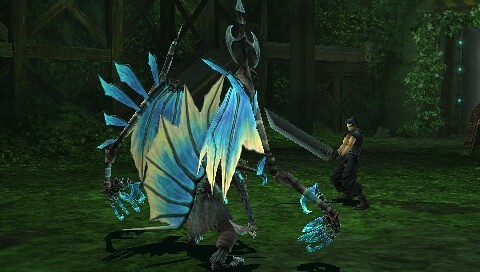A scene from a video game set in a lush clearing with dense woods in the background. In the center of the image stands a man with dark hair, dressed in an outfit that exposes his chest, black pants, and dark shoes. He holds a large silver knife with both hands, its blade gleaming menacingly as he adopts a combat stance with bent knees and a backward lean. In front of him, a piece of white cloth is stretched out and attached to a brown pole, which has additional strips of white fabric fluttering from it.